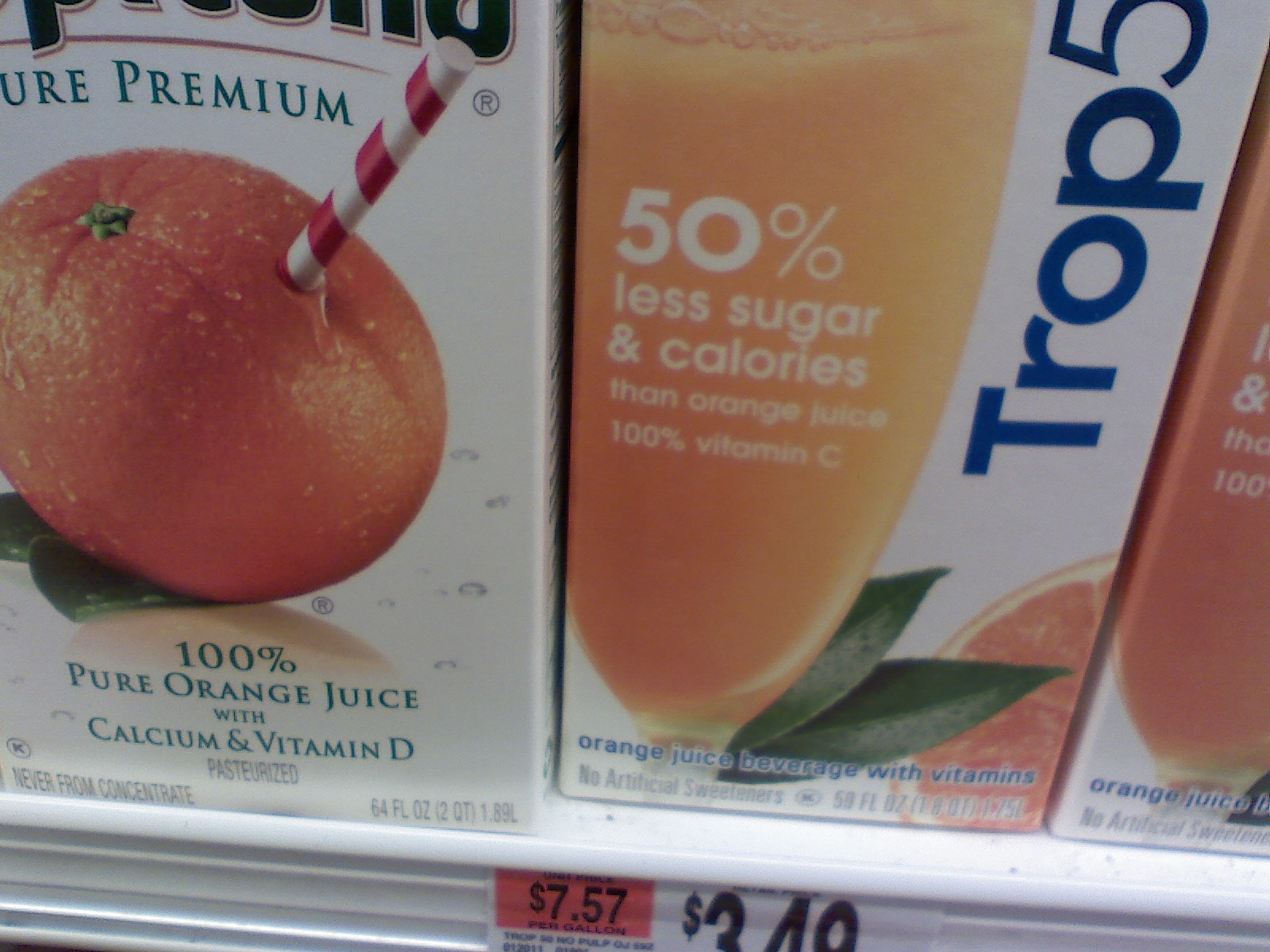The image showcases a product display for a premium orange juice beverage. At the center of the image, there's a picture of a whole orange with a straw sticking out of it, symbolizing the freshness and purity of the juice. Surrounding the central orange are various bubbles, enhancing the fresh and fizzy appeal of the beverage. 

The text on the image highlights a few notable features:

- The drink is labeled "100% Pure Orange Juice" with a mention of a consistent amount of Vitamin B.
- The caption reads "Never More Concentrated" and provides measurements of "64 fluid ounces" and "2 quarts (0.29 liters)."
- Additional text indicates "50% Less Sugar and Calories" and ensures the juice is "100% Vitamin C."
- It specifies that the orange juice is a "Beverage with Vitamins, No Artificial Sweeteners."
- Further details mention "9.4 ounces" and "1.8 quarts." 

An orange label at the bottom indicates a price of "$7.57," while a smaller label to the right displays "$3.49." Also, on the right side of the image, there's another glass of orange juice with frothy bubbles on top and some white and green leaves for decoration, reinforcing the natural and refreshing theme of the product. The words "Tropical Five" add a touch of exoticism, and the image also features orange slices and three leaves to further emphasize the natural ingredients.